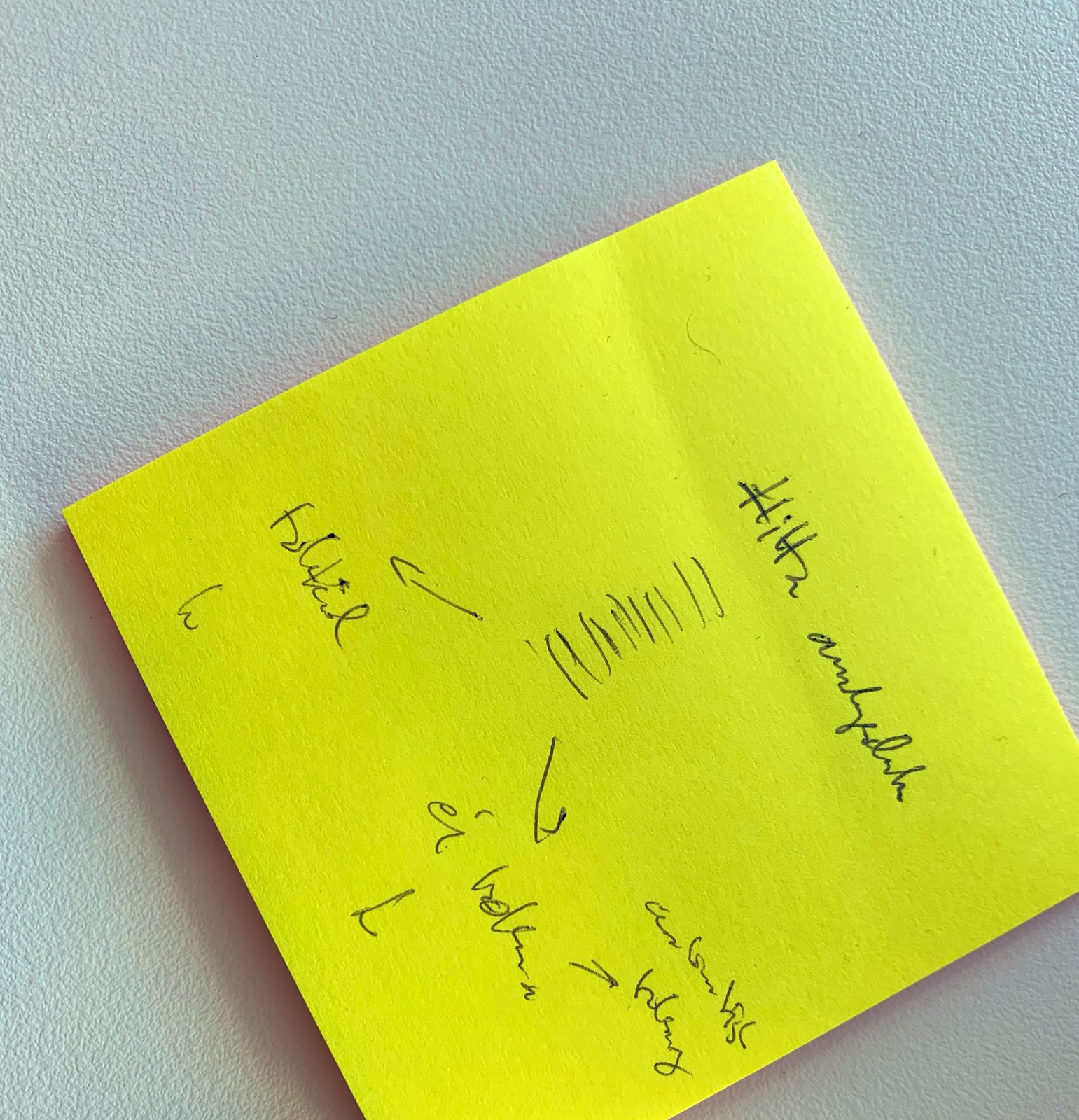The image features a close-up view of an off-white surface, showcasing its detailed textures, pores, and small dots. This monochromatic surface serves as the backdrop for a yellow square piece of paper, positioned at a diagonal angle across the image. The yellow paper appears to be a sticky note, adorned with indiscernible scribblings in a hurried and illegible handwriting. Among the markings, there are several short horizontal lines, accompanied by arrows. One arrow points to the left, while another directs attention to the right, creating a chaotic and enigmatic scene captured in minute detail.